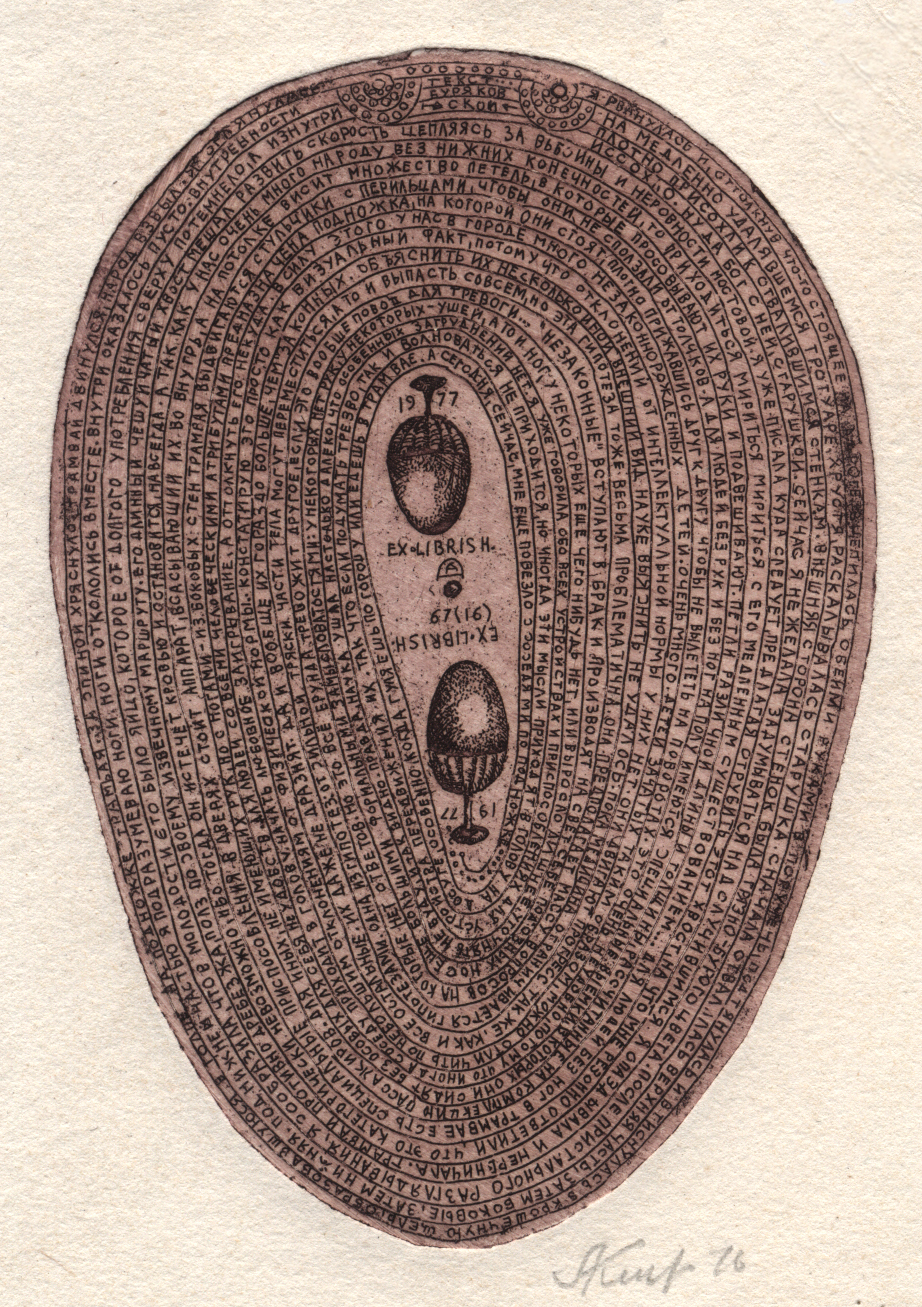The vertically rectangular image showcases an intricate drawing against a textured background that shifts between light gray and shades of white and brown. The main feature is a flat, egg-shaped oval, more rounded at the top than the bottom, filled with layers of spiraling lines and symbols. Central to this oval are two images resembling large eggs or wine glasses—one positioned upright at the bottom and the other inverted at the top. Both central figures are surrounded by extensive, unreadable writing and symbols. There is an inscription within the central area, marked with the numbers 1977. Toward the bottom right corner of the image, an artist’s signature starting with the letter 'K' is visible, likely followed by the year, possibly '76 or '16'. The piece appears to be rendered in darker brown ink, creating a prominent contrast against the lighter textured backdrop, and possesses an enigmatic, museum-quality aura.